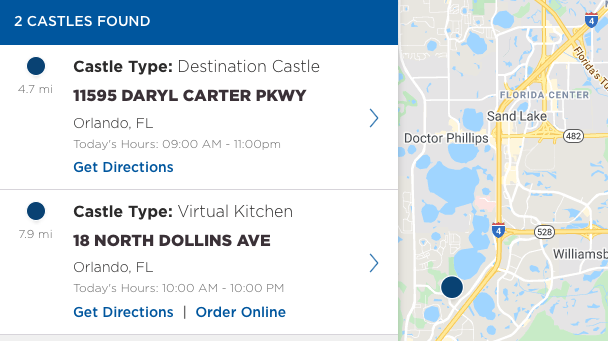This image is a cropped screenshot of the White Castle app. At the top left, the screen has a blue border with the text "Two castles found" in white font. Below this header, there are listings for two different White Castle locations, and to the right is a rectangular map that extends along the side.

For the first White Castle entry, on the left, there's a blue dot indicating the location is 4.7 miles away. To the right of this dot, the text reads "Castle type: Destination Castle" with the address listed below as 1595 Darryl Carter Parkway, Orlando, Florida. This entry also includes the information "Today's hours" followed by a blue link for "Get directions."

The second White Castle entry is similarly structured but labeled as a "Castle type: Virtual Kitchen." The address for this location is 18 North Dollins Avenue, Orlando, Florida. Like the first entry, it provides "Today's hours" along with options to "Get directions" and "Order online," with "Order online" highlighted in blue. The remainder of the web page is cropped out in the image.